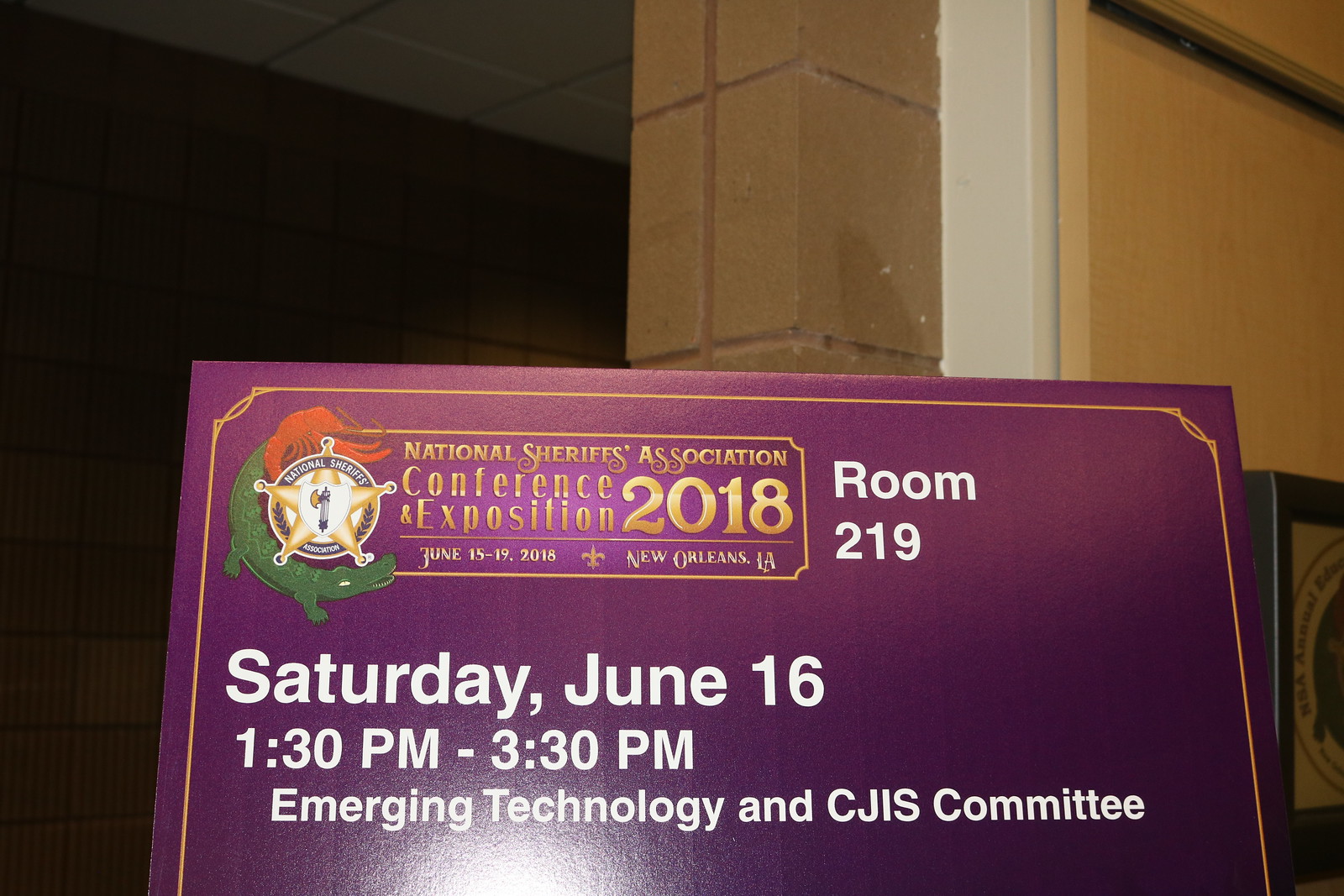This photograph captures a poster for the National Sheriff's Association Conference and Exposition 2018. The poster is positioned standing against a brick column in an older, dimly lit building, with a brown paneled wall on the right and lighter brickwork in the center background. The poster itself has a solid wine purple background accented with a golden border. Prominently displayed at the top of the poster in gold lettering is the event's name: "National Sheriff's Association Conference and Exposition 2018." Below this, the event dates "June 15-19, 2018" and location "New Orleans, Louisiana" are also highlighted. On the top left of the poster is the organization's logo, featuring a sheriff's star encircled by a green alligator and a red lobster. The poster provides further details about an event: "Saturday, June 16th, 1:30 p.m. to 3:30 p.m. Emerging Technology and CJIS Committee," held in Room 219, noted in bright white text. The flash used in the photograph creates a reflection on the sign, emphasizing its glossy finish and adding contrast to the overall dark and historic atmosphere of the setting.